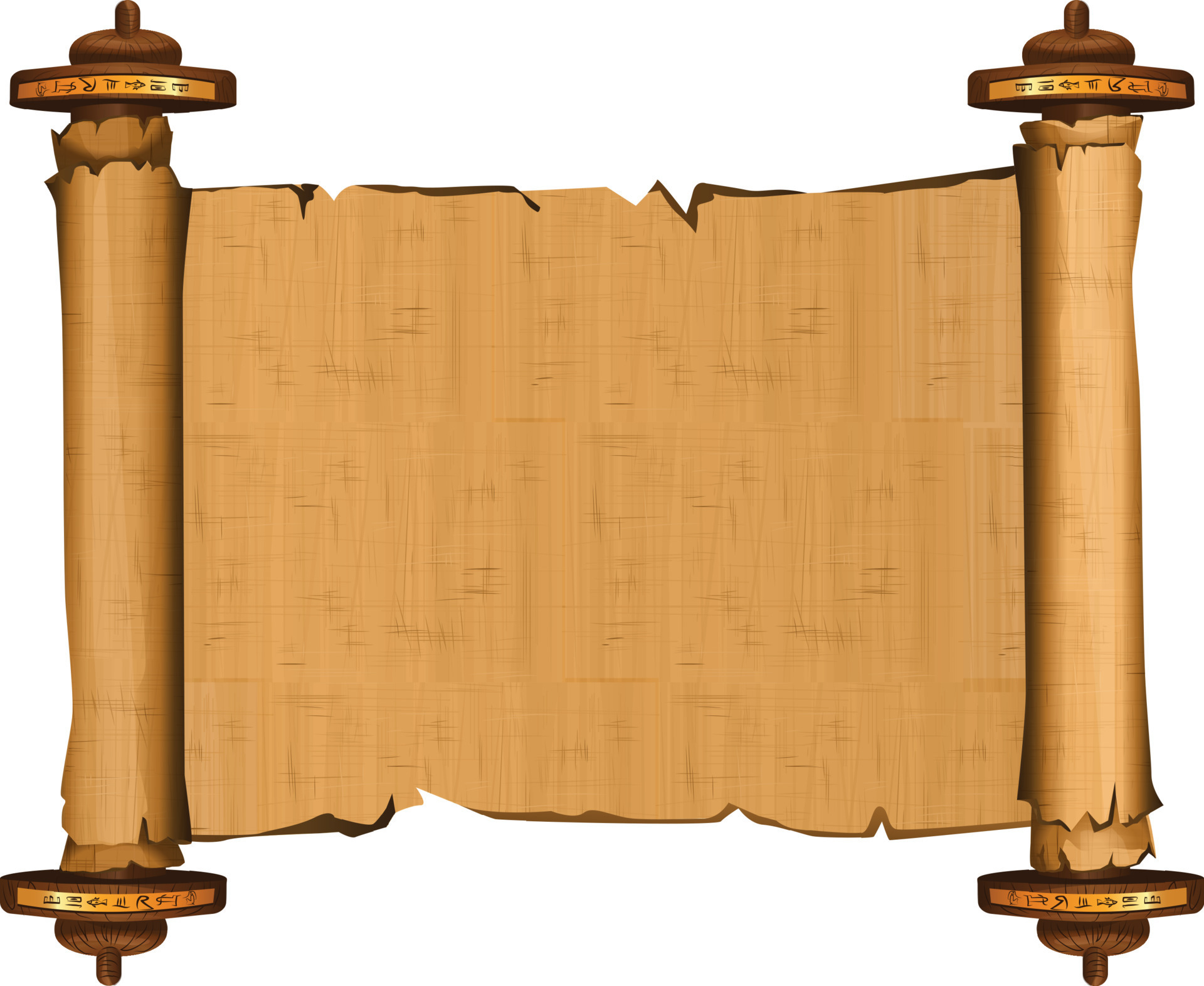The image is a detailed digital graphic of a wide-open scroll with two prominent handles on either side. The scroll itself is a tan-brown color, displaying worn textures with jagged, torn edges both at the top and bottom. These edges and the way the paper is unfurled from the handles convey an ancient, weathered appearance. Each handle, darker brown in colour, features a pointed top and bottom. The circular tops of the handles, adorned with intricate, hieroglyphic-like symbols in black ink bordered by golden lines, add an ornate touch to the design. The handles also possess an ornamental cylindrical object in the middle with a gold-patterned ring. Set against a white background, the scroll exudes an aura of antiquity, enhanced by the engravings and its detailed, aged aesthetic.